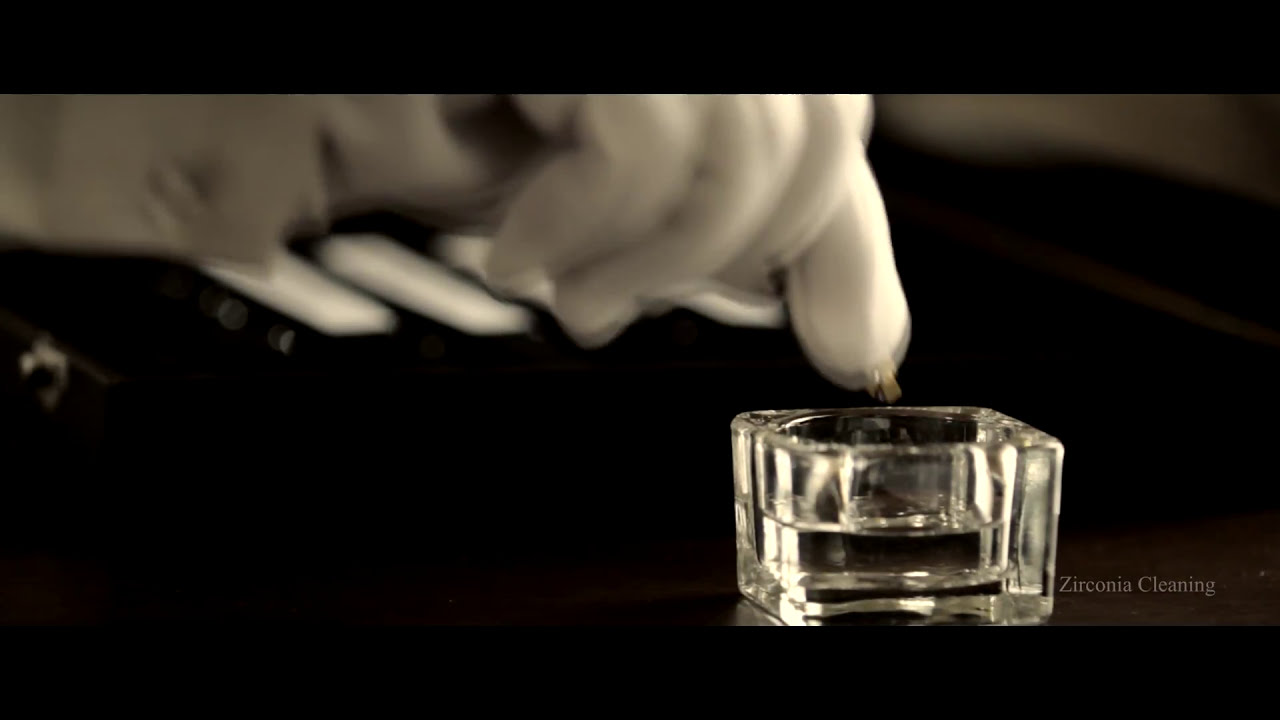This close-up photograph captures a scene focused on a small, thick-walled glass container holding a clear liquid, likely used for jewelry cleaning given the text "zirconia cleaning" in white lettering at the bottom right. The container, prominently featured and in sharp focus on a black surface, appears square with a circular indentation in the center. Hovering above the glass is a blurred, motion-captured white-gloved hand, suggesting an action of dipping into the liquid. The background is heavily blurred with subtle hues of brown and black, making the glass container and glove the central elements of the image. Additionally, three white piano keys are faintly visible in the background, adding a touch of context to the setting.